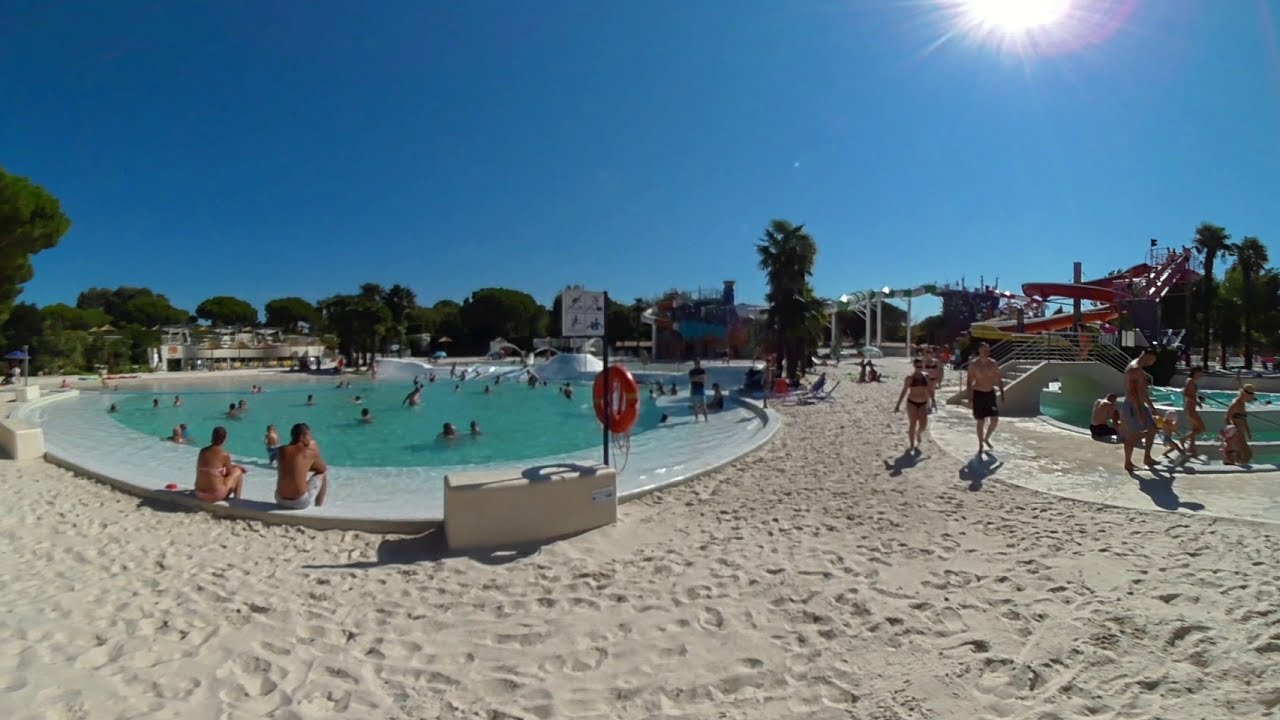The image depicts a lively outdoor water park with sandy paths surrounding various structures. To the left, a large, round pool with blue-green, chlorinated water is filled with many swimmers. Two people—one woman in a bathing suit and a shirtless man—sit at the edge of the pool, their backs to the viewer. On the right side, there's another pool, possibly a lazy river, with a red and yellow water slide above it. People in swimsuits walk along the sandy paths and sit by the edges of the pools. In the foreground, a sandy area stretches across the image, giving way to more sandy paths between the pools. In the distant background, tall green trees frame the scene along with a building on the left and various structures on the right, including what appears to be another larger tube slide. The sky above is clear blue, with the sun shining brightly in the upper right-hand corner of the image.